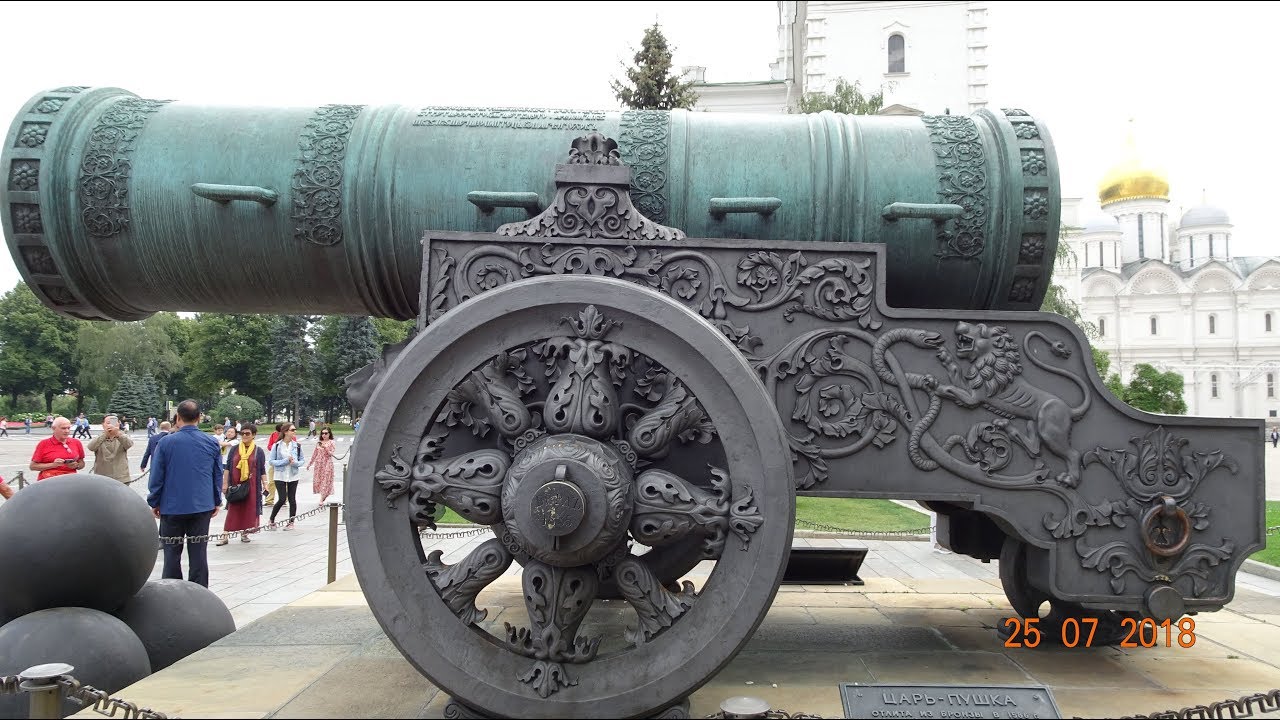In this outdoor image, you are greeted by a striking display of a massive, teal-colored cannon adorned with intricate engravings and four side handles. The cannon's barrel rests on a grand, black iron base featuring ornate designs of lions, snakes, and vines. It includes a giant wheel with an intricate owl-like design. A trio of black cannonballs lie beneath the front of the cannon. To the left, groups of people observe and photograph the impressive artifact. In the background, beyond a row of lush green trees, you see a two-story white building with a gold-topped tower against a pale, clear sky. The bottom right corner of the picture is marked with the date "25072018," alongside a sign in a non-English language.